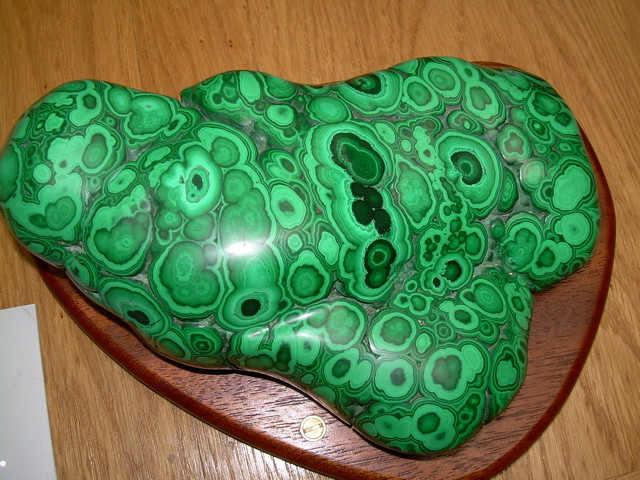This square image features a wooden surface that might be a wood tile, table, or countertop, characterized by a medium brown color with slightly darker grain patterns. At the center of this background is a dark, heart-shaped wooden object, possibly a cutting board or plaque. Dominating this object is a large, irregular, and bumpy shape with a green patterned surface. The intricate design showcases various shades of green, ranging from light to very dark. This shape, which might resemble an inflatable pillow but also suggests polished rock or porcelain, boasts a stylized green pattern of irregular blobs. The textured surface appears raised in parts, adding depth to the object. In the lower left-hand corner, a part of a paper edge is visible, adding a subtle detail to the composition.